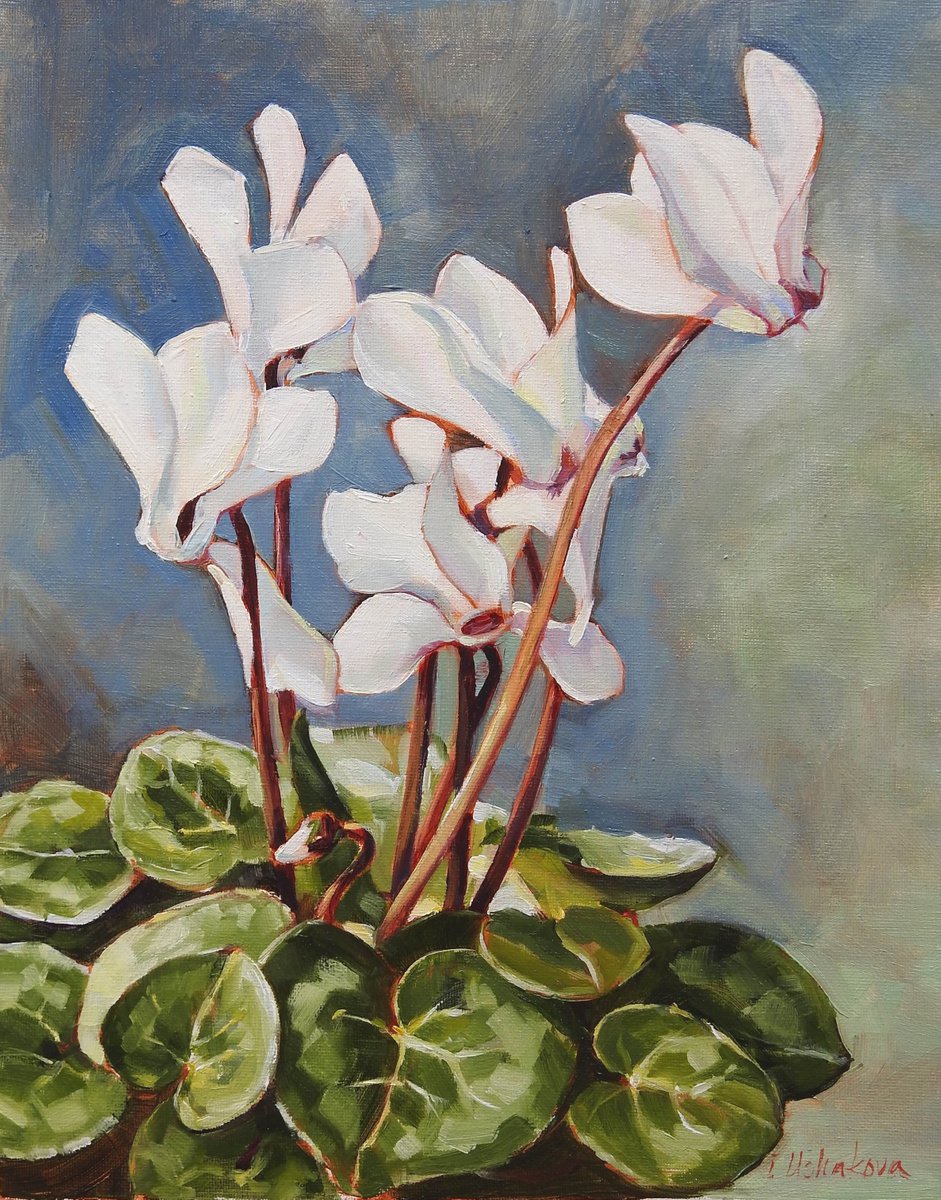This painting, reminiscent of Monet’s impressionistic style, features six elegant white lilies gracefully perched on brown stems, rising from a lush cluster of heart-shaped green leaves. The foliage displays a spectrum of greens, darker on the periphery and lighter towards the center. The background blends soothing hues of blues and greens with occasional touches of white and yellow, adding to the serene ambiance. The large petals of the flowers, which appear to sway softly in an unseen breeze, dominate the top middle section of the painting, while the verdant leaves fill the lower portion. The detailed brushstrokes are clearly visible, enhancing the painting's tactile quality. In the lower right-hand corner, the artist has signed their work with a light red inscription that reads "I. Ushakova," adding a personal touch to this vertical masterpiece.